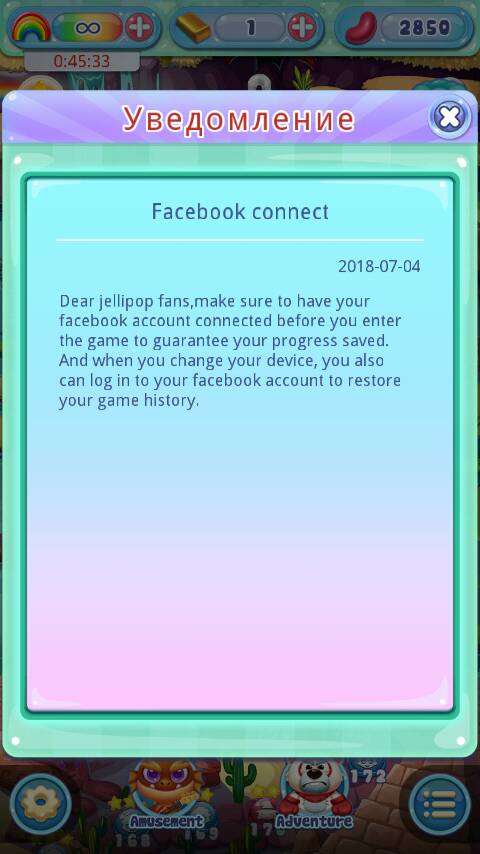The image is a screen capture from a mobile game that has a cartoonish style, reminiscent of Candy Crush, called "Jelly Pop." The background of the screenshot is slightly tinted out, making it hard to see the game clearly. However, visible elements include player stats like a score of 2850 in the upper right corner, a gold bar icon with the number 1 next to it in the upper-middle section, and a rainbow-colored oval with an infinity sign in the upper left.

Dominating the screen is a pop-up notification window with a purple headline featuring red Cyrillic lettering, likely Russian. The main message, set against a teal box, reads: "Dear Jelly Pop fans, make sure to have your Facebook account connected before you enter the game to guarantee your progress is saved. When you change your device, you can also log into your Facebook account to restore your game history." The notification also includes the date "2018-07-04" on the right, along with a white X in the upper right corner to close the message. Behind the pop-up, a settings symbol can be seen in the bottom left, and a menu symbol in the bottom right corner.